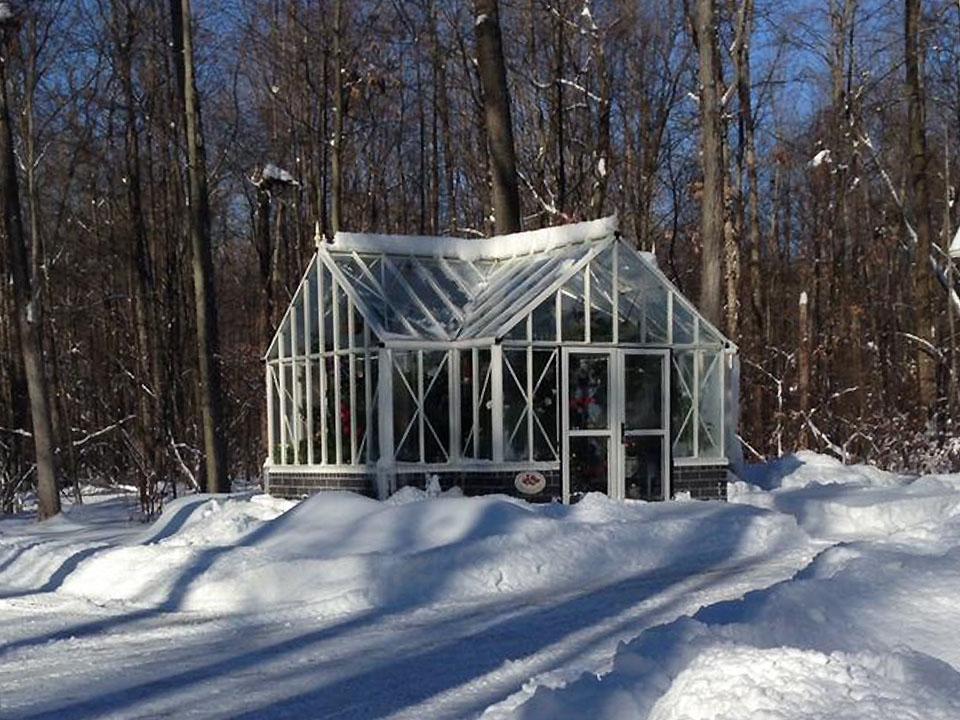In this late afternoon, countryside scene, a snow-covered landscape sets the stage for a detailed photographic image. The centerpiece is a distinctive greenhouse made of metal and glass, situated amidst a heavily wooded area. The greenhouse, shaped like an L with a gabled roof, stands out with its intricate structure of metal poles supporting clear, reflective windows. Snow blankets the foreground, and the shadows of tall, bare trees stretch elegantly across the pristine white ground. The trees, mostly leafless with a few retaining brown leaves, frame the scene against a backdrop of a clear, cloudless blue sky.

At the forefront of the greenhouse, there's a small emblem next to a set of double doors, though the text on it is unreadable. The greenhouse's lower part features gray brick, and a sign with white and red text, too distant to decipher, adorns the front. Inside the greenhouse, various trees, bushes, and possibly flowers thrive, creating a lush contrast to the winter exterior. A carefully shoveled trail leads up to the greenhouse, suggesting a maintained path through the deep snow. This visually rich image encapsulates a serene, wintry afternoon in the countryside, merging natural beauty with human craftsmanship.